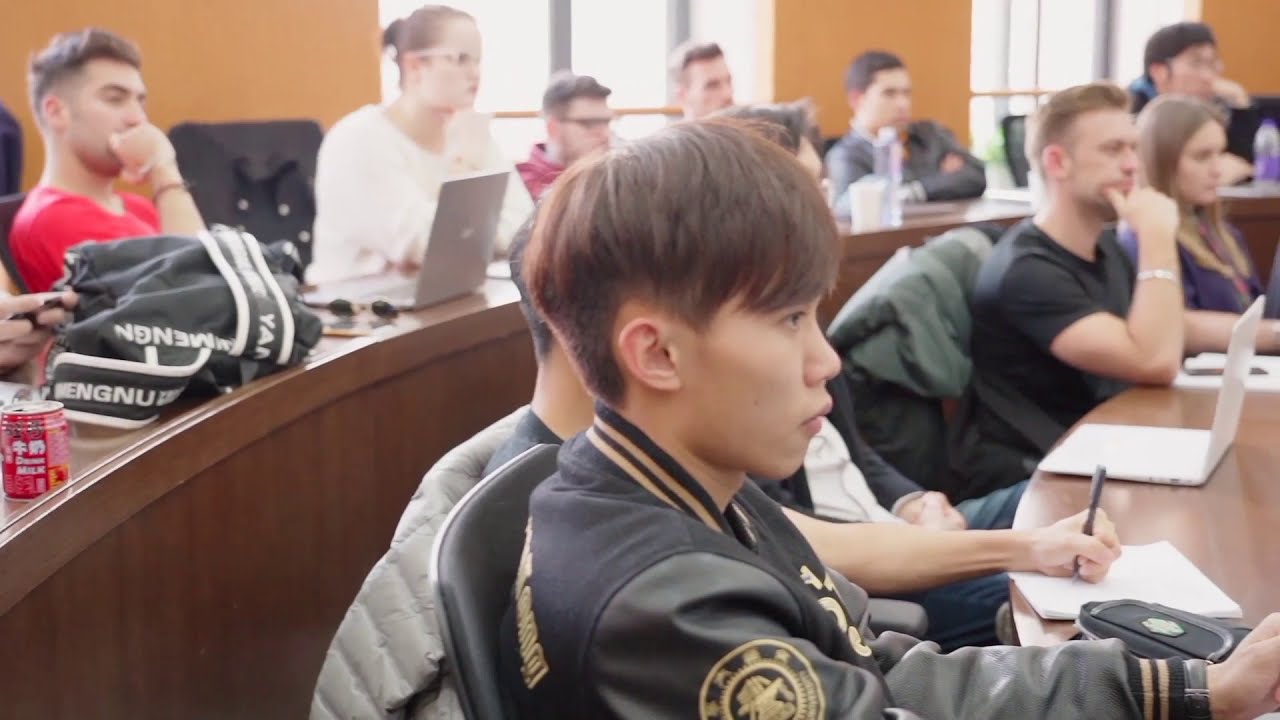The photograph depicts a college classroom filled with engaged students, likely young adults. The classroom features a wide, rectangular layout with two visible rows of long wooden desks forming a curved, circular seating arrangement. The walls are painted orange, accentuated by giant white windows with black panes, casting natural light into the room. The desks are brown and spacious, adorned with a mix of open tablet devices and traditional pen and paper. 

Front and center, a young Asian male with short brown hair wears a distinctive black jacket with gold accents. Around him, students are actively participating in the lesson, taking notes and listening attentively. In the background, among the diverse group, a man with reddish facial hair wears a black t-shirt, while nearby, another student in a red shirt and a girl in a white shirt with glasses attend the class. On a distant desk, a red can and a black bag can be spotted, adding subtle detail to the busy educational environment. The colors in the room are varied and vibrant, including black, white, yellow, red, gray, gold, purple, and brown, contributing to a lively learning atmosphere.